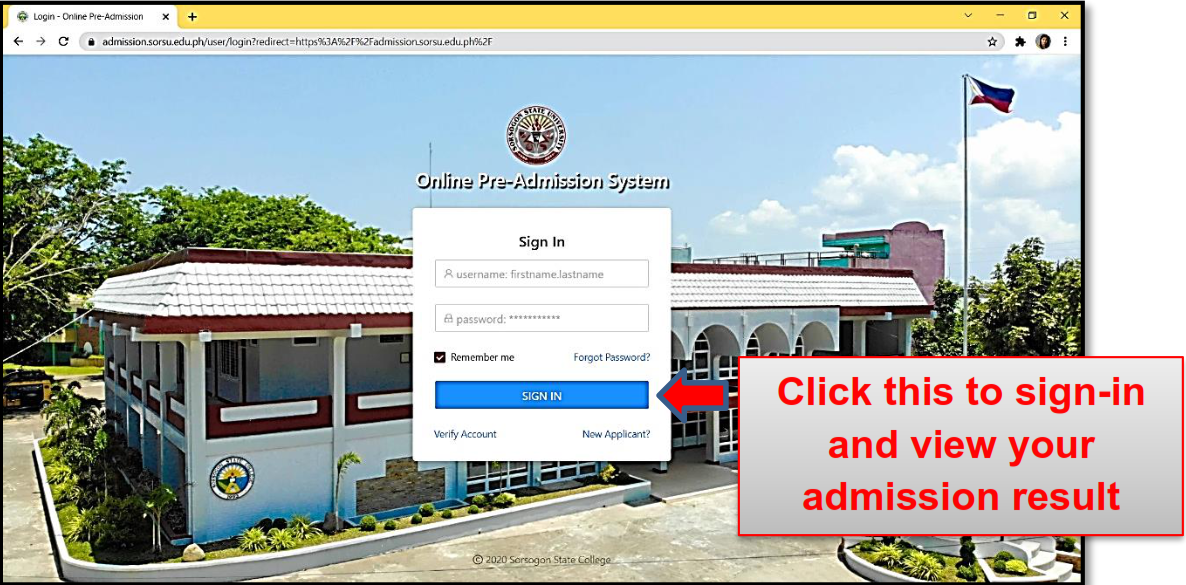The image depicts a portion of a website. The central part of the image focuses on a two-story building with white walls. The building features multiple large, arched windows and arched doorways on the ground floor. The roof is flat, with a portion of it slightly slanted, covered in white tiles. A balcony is visible on the second floor on the left side, with doors leading onto it. There's a circular emblem on the building displaying blue and yellow colors, although the text within it is not readable.

The exterior section of the image shows a concrete parking lot with a visible flagpole that raises a flag in blue, red, and white. The surrounding landscape includes trees and bushes, and there is a partially obscured object that could be a fountain. The sky above is clear and blue.

Above the building, in the website interface, there is a yellow banner, under which is a white bar designated for search functionality. This section contains the name of the website, although the text is too small to discern. 

At the top of the image, a white square area indicates instructions for an "Online Pre-Admission System" with text fields for entering a username and password, along with a 'Sign In' button. Additionally, at the bottom right, there is a rectangular section outlined in red that instructs users to click to sign in and view their admission results.